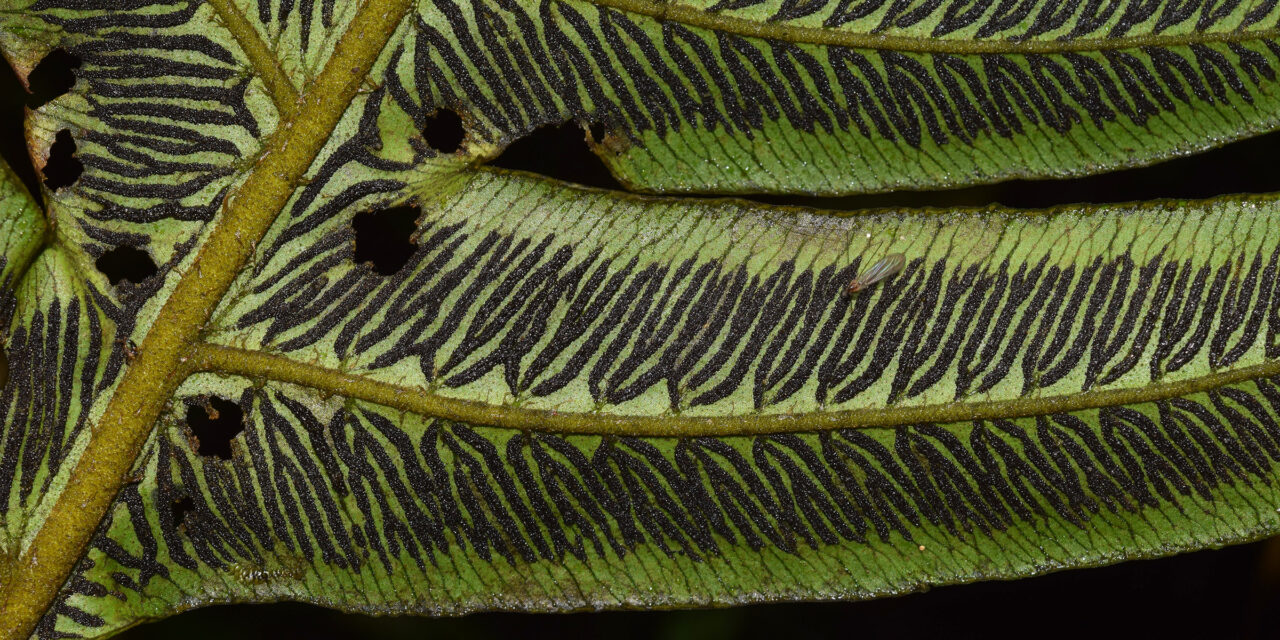This image captures a very close-up and highly detailed view of a leaf against a black background, arranged in a horizontal rectangular frame. Emerging from the bottom left corner and ascending at a slight angle to the top, a light green stem splits into several thinner stems. These stems support long, triangular leaves seen from their underside. The leaves are a light green and feature vertical black lines that originate at the edges, starting as thin and light but becoming thicker and darker as they approach the leaf center. The large, dark green main stem stands out on the left, branching off to the right into wide, elongated leaves, with the most prominent leaf extending towards the right. The leaves appear to have been partially eaten, marked by significant holes, especially on the left side of the image, suggestive of insect activity. A long-winged insect is also visible in the upper central part of the leaves.